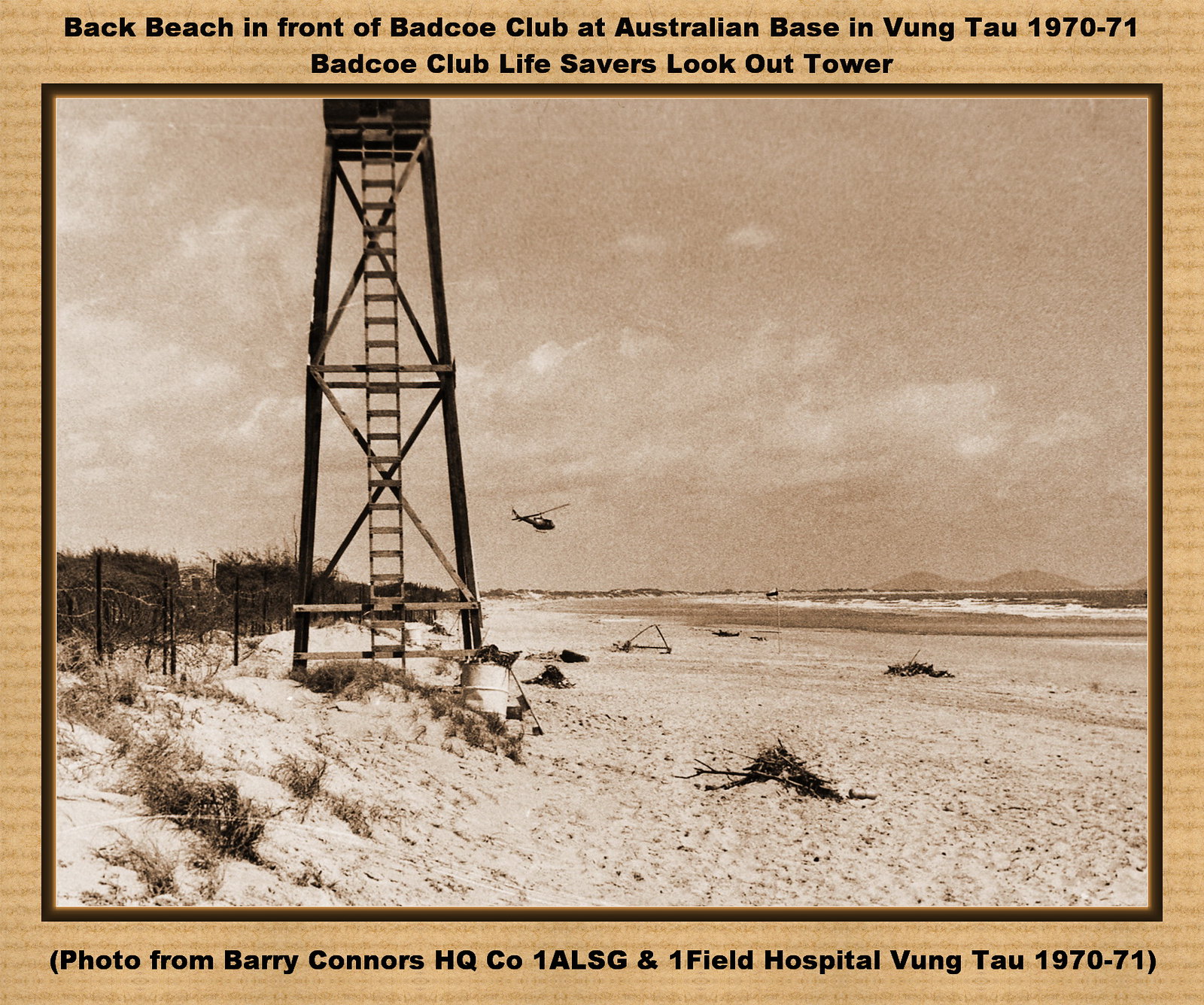This sepia-toned black and white photograph, taken outdoors during the daytime, captures a serene yet historically significant scene at Back Beach, in front of the Bad Co. Club at the Australian base in Vung Tau, during 1970-71. The photo, bordered by a textured light brown frame with a darker brown outline reminiscent of wood or cardboard, was taken by Barry Connors from HQ Company, 1ALSG, and One Field Hospital.

In the foreground, beach grass and barbed wire fencing accentuate the sandy beach that stretches toward the water on the right. Prominently on the left, there is a tall wooden lifesavers lookout tower with a ladder reaching to the top. Near the tower, partially concealed by the beach grass, additional fencing can be seen, adding to the militaristic ambiance. Dominating the upper portion of the image are a cloudy sky and distant mountains on the horizon. Centrally positioned and capturing attention, a black helicopter hovers low, flying towards the shore. The blend of these elements evokes a glimpse into the historical era of the location.